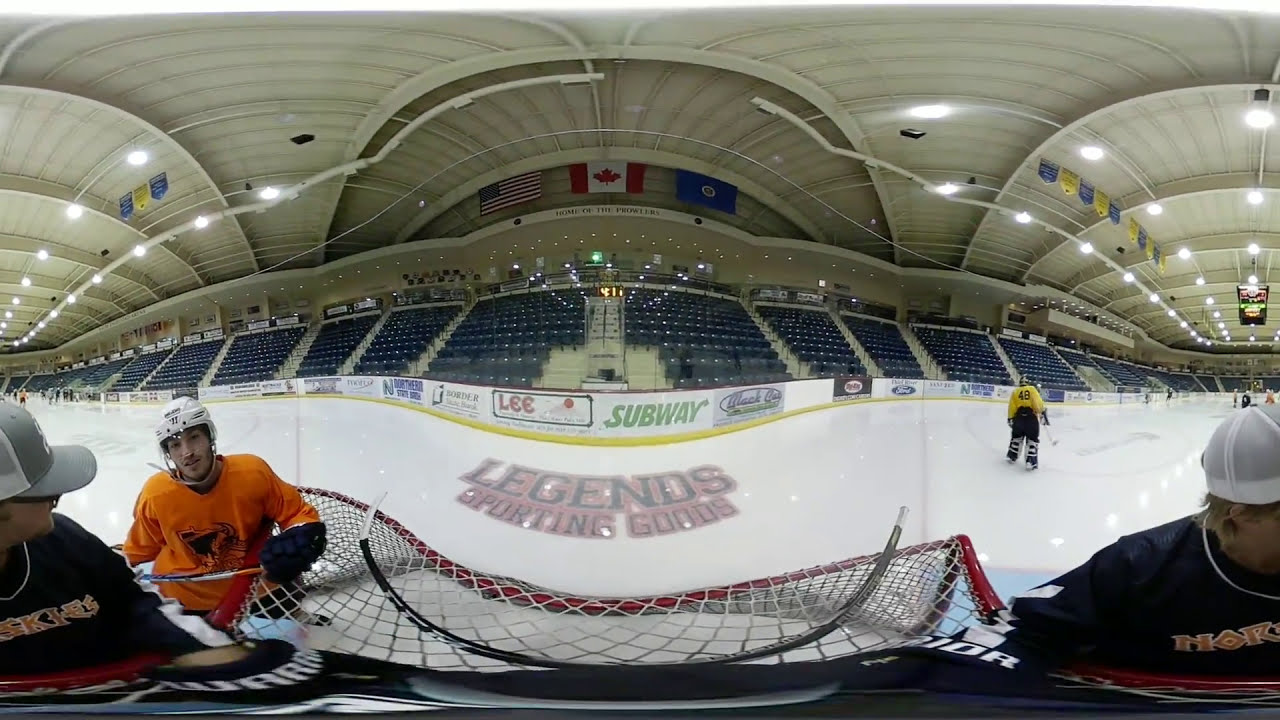This is a dynamic fisheye view photograph of an indoor ice hockey stadium capturing a live game. The image, taken from the middle of the rink, features text reading "Legends Sporting Goods" prominently displayed on the ice. The stadium foreground shows a player in a white helmet wearing a pink jersey and holding a hockey stick. The central figure appears split, suggesting the photograph was taken using a fisheye lens or filter, resulting in a curved and distorted effect.

In the left corner, another player is seen in a bright orange full-sleeve jersey, equipped with gloves and a stick, standing by the goal post. The player faces a fan who wears a cap, spectacles, a black t-shirt with a white wire or chain around his neck. Nearby, another individual with blonde hair, wearing a dark blue t-shirt partially showing the text “N.O.R.” and a white wire, adds to the scene's activity.

The background reveals a nearly empty audience gallery with blue chairs, multiple hanging banners, and illuminated ceiling lights. Three national flags, including those of the USA and Canada, hang near the roof, with the text "Home of the Prowlers" visible above. Several advertisements from sponsors such as Lee and Subway line the stadium's boundary walls. Farther back on the right side, players in yellow and various other colored jerseys, including number 48, are seen, along with a scoreboard suspended from the ceiling.